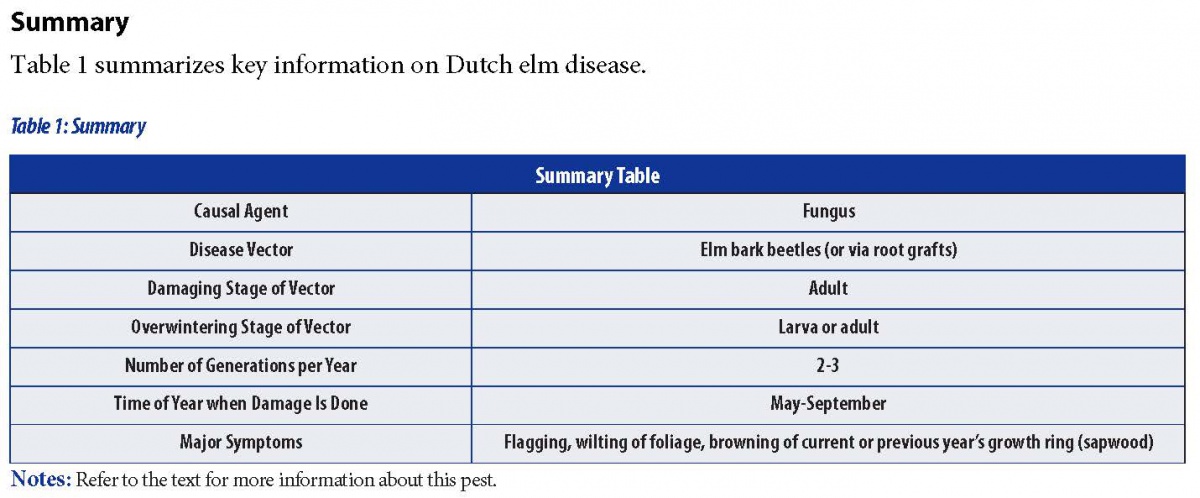The image displays a detailed summary table (Table 1) on Dutch Elm Disease against a white background. At the top is a black-font title reading "Summary." Below this, a dark blue heading with white font states "Summary Table." The table is structured with seven rows and two columns. The first column provides categories: "Causal Agent," "Disease Vector," "Damaging Stage of Vector," "Overwintering Stage of Vector," "Number of Generations per Year," "Time of Year when Damage is Done," and "Major Symptoms." Corresponding entries in the second column include: "Fungus," "Elm Bark Beetles or Via Root Grafts," "Adult," "Larva or Adult," "2-3," "May-September," and "Flagging, Wilting of Foliage, Browning of Current or Previous Year's Growth Ring, Sapwood." At the bottom, a notation reads, "Refer to the text for more information about this pest."